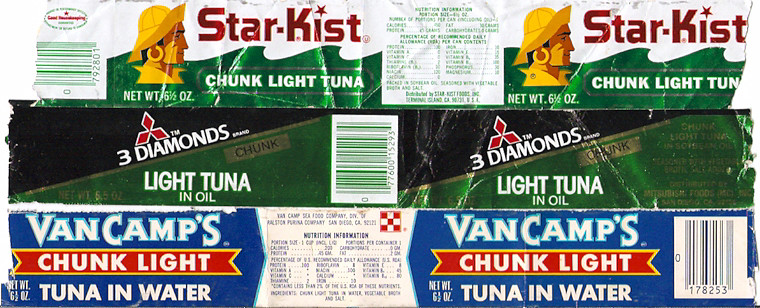The horizontal image captures the intricate details of a Starkist Chunk Light Tuna can label. The label wraps around the can, displaying identical information on both the front and back. 

At the top of the label, a fisherman is depicted in profile, accompanied by the Starkist logo in red. The product name, "Chunk Light Tuna," appears in white on a green wave beneath the fisherman. 

The central portion of the label features a barcode, flanked by a distinctive logo with three diamonds aligned at an angle, alongside the text "Light Tuna in Oil" in both white and red lettering.

The bottom section showcases a partially blue label with white lettering, including the Ralston Purina mark. Nutritional facts are centered prominently. The phrase "Van Camp's Chunk Light Tuna in Water" is displayed in white letters against a blue background, with "Chunk Light" highlighted on a red banner. The barcode is positioned at the far right end of this segment.

This detailed label design provides a comprehensive display of the product's branding, nutritional information, and company affiliation.